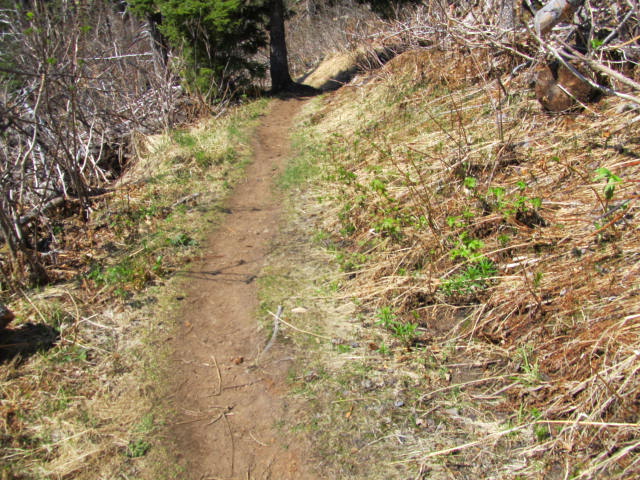A barren forest trail winds through a landscape that appears to be recovering from a wildfire. The ground is sunlit, casting a pronounced shadow from the sole tree visible in the distance. Surrounding the trail, only sparse bushes and weeds punctuate the empty, desolate terrain. The trail itself is flat and devoid of any footprints, suggesting it is seldom traveled. The right side of the scene is distinctly more elevated than the left, adding a subtle tilt to the barren landscape. No people or wildlife are present, enhancing the scene's sense of isolation and recovery.